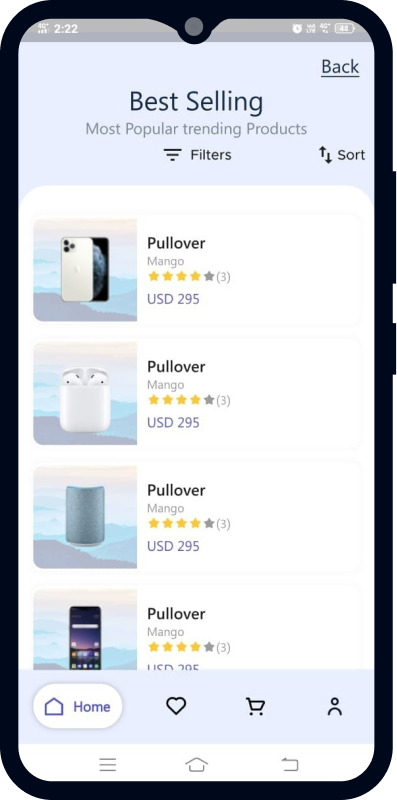This photo showcases a mobile phone displaying an online shopping app. The phone screen is bordered by black on the left and right sides, while the top border dips approximately half an inch and then rounds back up, with a small gray dot in the center of this dip. On the left side of the gray dot, there is a gray border and on the right, the time "2:22" is displayed within a gray border. The phone's battery status shows 48%, alongside the indicator "4G LTE" and an active alarm clock icon.

Below the status bar, the screen features the app's header with prominent black text. First, there is a large title "Best-Selling" with smaller, bold lettering underneath stating "Most Popular Trending Products." Below this header, three progressively smaller lines appear on the left side indicating a tab or menu, while on the right side, there is an option labeled "Filters" next to small black up and down arrows accompanying the "Sort" function.

The main content area displays product listings, focusing on phones. Four phone images are aligned vertically along the left side, each with corresponding product names, star ratings, and prices on the right side. This section has a white background and extends to about two inches from the bottom of the screen.

At the bottom, a blue border separates the main content from the navigation bar. The navigation bar features white tabs with icons and text labels: a home icon with "Home," a heart icon for favorites, a shopping cart icon, and an account icon. Beneath the navigation bar, in the white section, there are three parallel lines on the left, another home icon, and a line running across the bottom of the screen from right to left, ending with a small arrow on the left side.